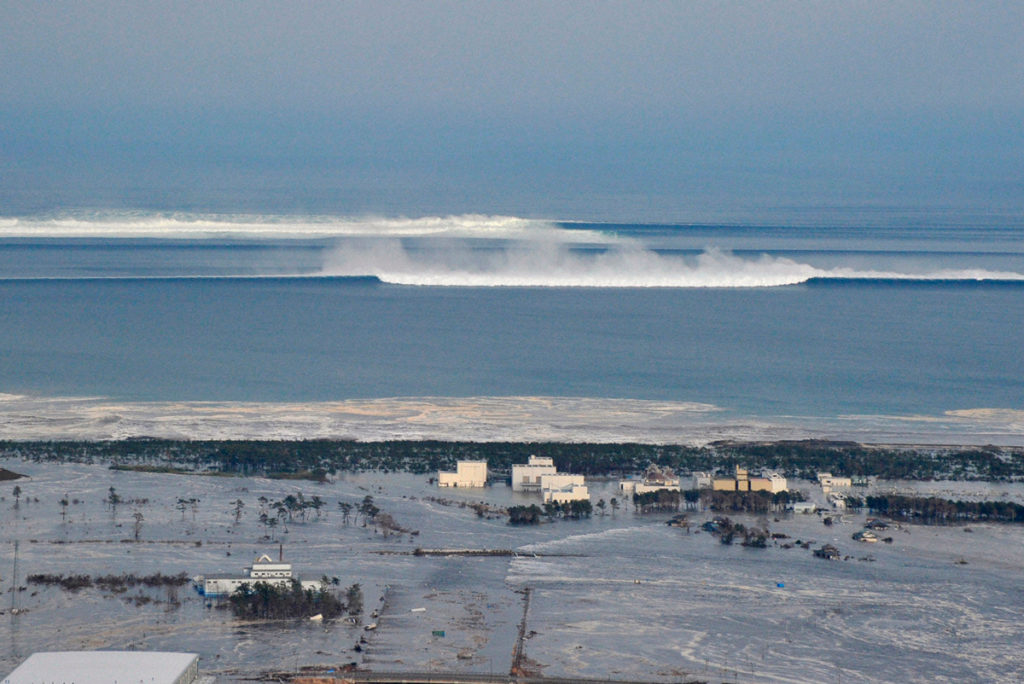This aerial, photorealistic image captures a coastal scene that appears to be taken during the day under a clear, blue sky. The horizon shows large waves crashing against the shore, possibly indicating a recent storm or tsunami. The vast ocean spans the entire width of the photo, with waves forming a noticeable boundary.

Moving towards the land, the scene reveals a town severely impacted by the water. The landscape is dominated by floodwaters, submerging cars, houses, and trees—only the treetops are visible above the waterline. The collection of buildings is faint and far off, so much so that their exact nature—whether they are houses, an airport, an offshore drilling rig, or even an Alaskan shopping mall—is indistinguishable. Despite the lack of clear details, the structures are evidently water-damaged and likely abandoned due to evacuation.

This detailed, zoomed-out perspective emphasizes the vastness and severity of the flooding, giving a sense of the widespread impact on the coastal area.